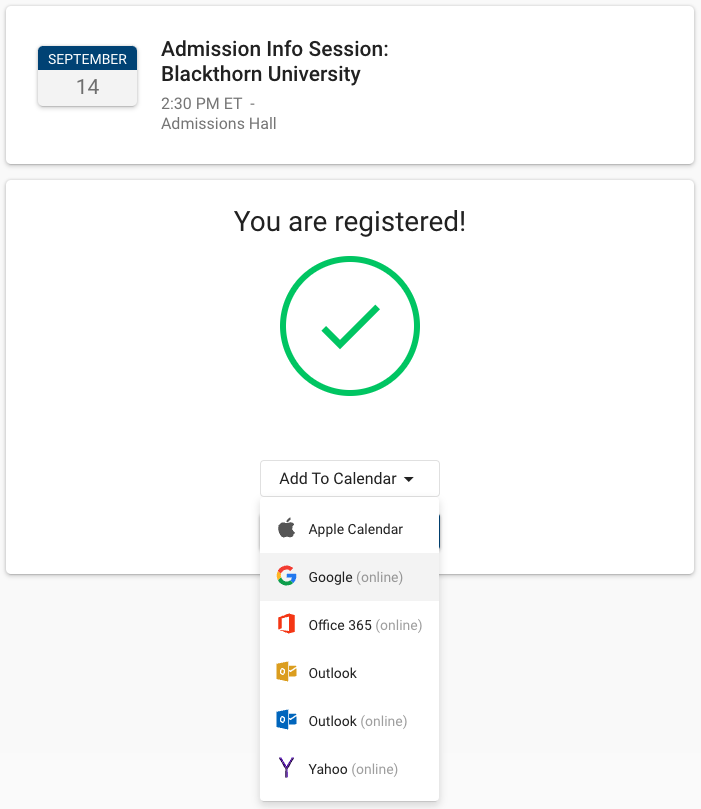The web page displays detailed information confirming a registration for an event. The interface is structured neatly with two prominent white boxes. 

The top box contains a calendar icon with a blue header indicating the current month - "September," and a grayish lower section featuring the date, "14." To the right, there is descriptive text in black font that reads:
"Admission Info Session
Blackthorne University
2:30 p.m. ET - Admissions Hall"

Below this, in a larger font, there's a confirmation message in white: "You are registered!" This is emphasized with a green circle containing a green checkmark. Below this message is a dropdown menu labeled "Add to Calendar."

The dropdown menu offers various calendar integration options including:

- Apple Calendar (indicated by the Apple logo)
- Google Calendar (indicated by the Google logo, with "Google" highlighted)
- Office 365 Calendar (indicated by the Office 365 logo)
- Outlook Calendar (indicated by the Outlook logo)
- Yahoo! Calendar (indicated by the Yahoo! logo)

Each entry allows users to seamlessly add the event to their preferred calendar platform. The overall page clearly confirms the registration for the event and provides multiple options to add the event details to various digital calendars.